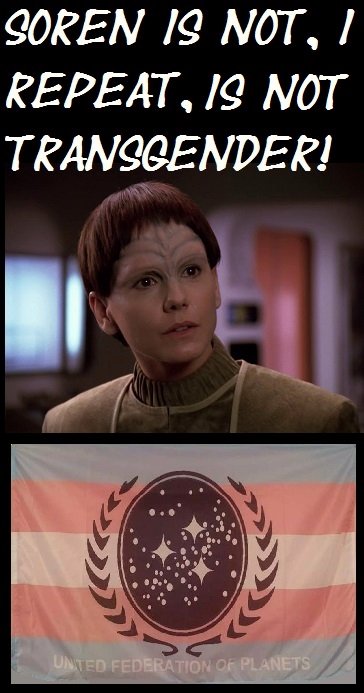This image is a vertical, portrait-style online meme divided into three distinct sections. The top section features white text on a black background that reads, "Soren is not, I repeat, is not transgender," explicitly clarifying the character's gender identity. The middle section contains a screen capture likely from a sci-fi TV show, possibly Star Trek. The character, named Soren, has short hair styled in a brunette bowl cut and sports outer space-themed attire, reminiscent of traditional Star Trek uniforms. The character's forehead has distinctive ridges and patterns, featuring two downward-pointing triangles, adding to their otherworldly appearance. Soren looks to the right, minimal makeup accentuating their alien features. The bottom section shows the flag of the United Federation of Planets, comprised of five horizontal bands in the colors blue, red, white, red, and blue. At the center of the flag is a circular emblem depicting stars, representing the galaxy, encircled by intricate filigree resembling leaves.